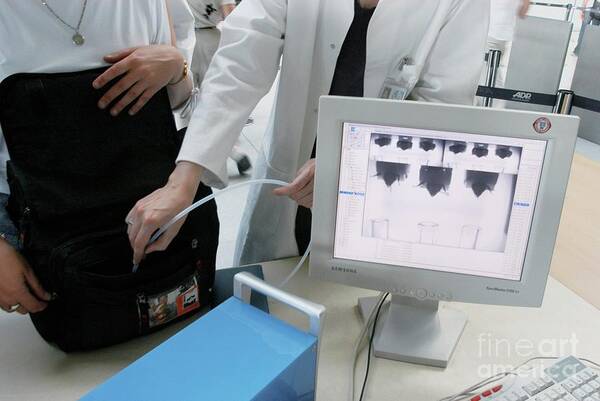In what appears to be a medical office or laboratory setting, the image captures a detailed scene involving two people. The person on the right is donned in a white lab coat, identifiable by a visible medical ID badge and a black shirt underneath. This individual holds a clear tube, which is inserted into a black bag held by the second person on the left, who is wearing a white shirt and a silver necklace. Although the content of the bag isn't visible, the setup hints at a medical procedure, possibly dialysis. The foreground features a computer monitor displaying a black-and-white image, which might be related to the tube's contents or a medical scan. Adjacent to this, part of a white keyboard and a bright blue box with a white handle can be seen, although the box lacks any discernible labeling. The background of the image reveals some barely legible lettering and various pieces of lab equipment, adding to the clinical atmosphere. Wires near the keyboard suggest connectivity to additional devices, reinforcing the technical and medical nature of the setting.